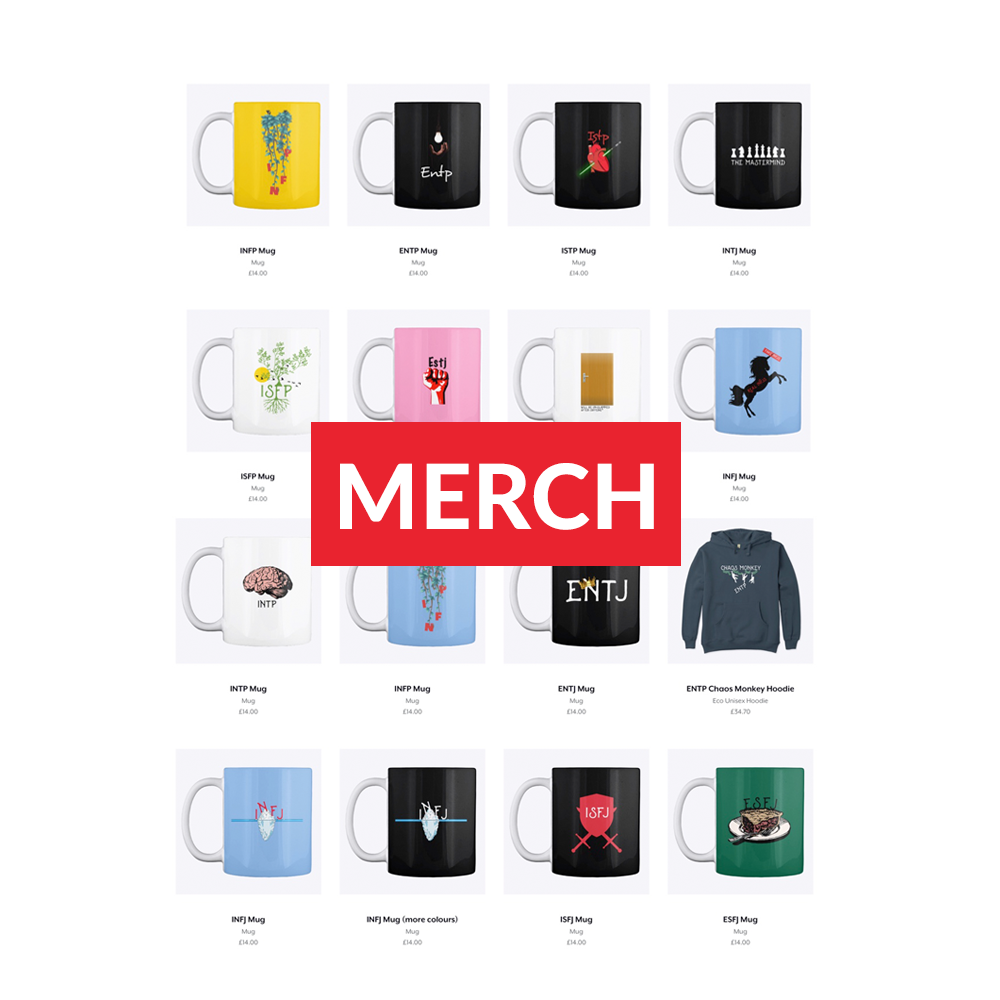A screenshot captures a shopping page featuring various merchandise items, predominantly focusing on mugs, with one exception being a hoodie sweatshirt. The store name is not specified, but a red rectangle with white text reading "Merch" is prominently displayed across the middle of the page. The assortment includes 16 distinct mugs and a single grey hoodie sweatshirt.

The mugs presented are as follows: 
1. A yellow mug adorned with a floral design.
2. A plain black mug.
3. A black mug featuring a red rose.
4. Another black mug with indistinct white figures.
5. A white mug with green leaf patterns.
6. A pink mug displaying a closed fist.
7. A white mug with a brown rectangle.
8. A light blue mug outlined with an animal figure.
9. A white mug showcasing an image of a brain.
10. A light blue mug with floral decorations.
11. A black mug inscribed with "ENTJ".
12. A light blue mug illustrating birds perched on a line.
13. A black mug depicting the same birds-on-a-line motif.
14. A black mug with a design resembling a sword crest.
15. A green mug potentially featuring a piece of pie.

Each item is captured in a thumbnail image, providing a visual overview of the merchandise available for purchase on this page.